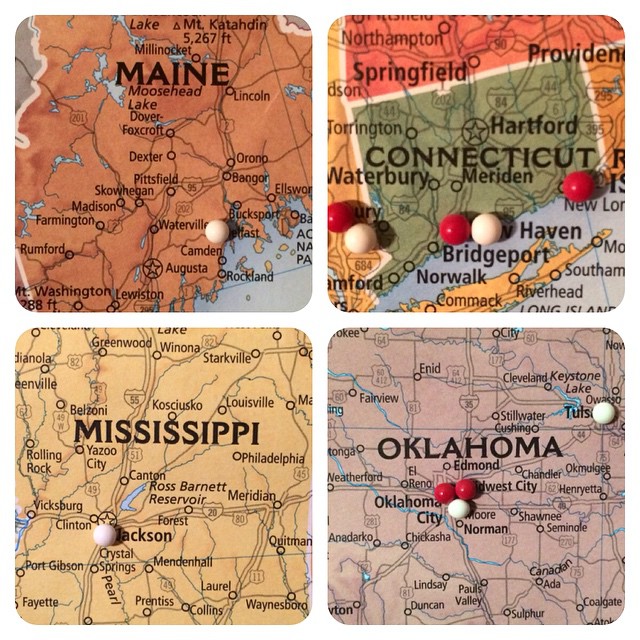In this image, we see a picture divided into four quadrants, each highlighting a detailed map of a different US state. The upper left quadrant features Maine, distinctively colored in orange/bronze. Various towns such as Moosehead, Lincoln, and Bangor are marked, with a noticeable white pin located near Camden. The upper right quadrant displays Connecticut in green, showcasing cities like Hartford, Waterbury, and Torrington, and marked with six pins in red and white. The lower left quadrant presents Mississippi in a beige hue, including cities like Louisville, Starkville, and Greenwood, with a white pin situated on Jackson. The bottom right quadrant illustrates Oklahoma in a rusty pink color, highlighting cities such as Edmond, Norman, and Oklahoma City, marked by four pins—including a white one near Tulsa and others around Oklahoma City.